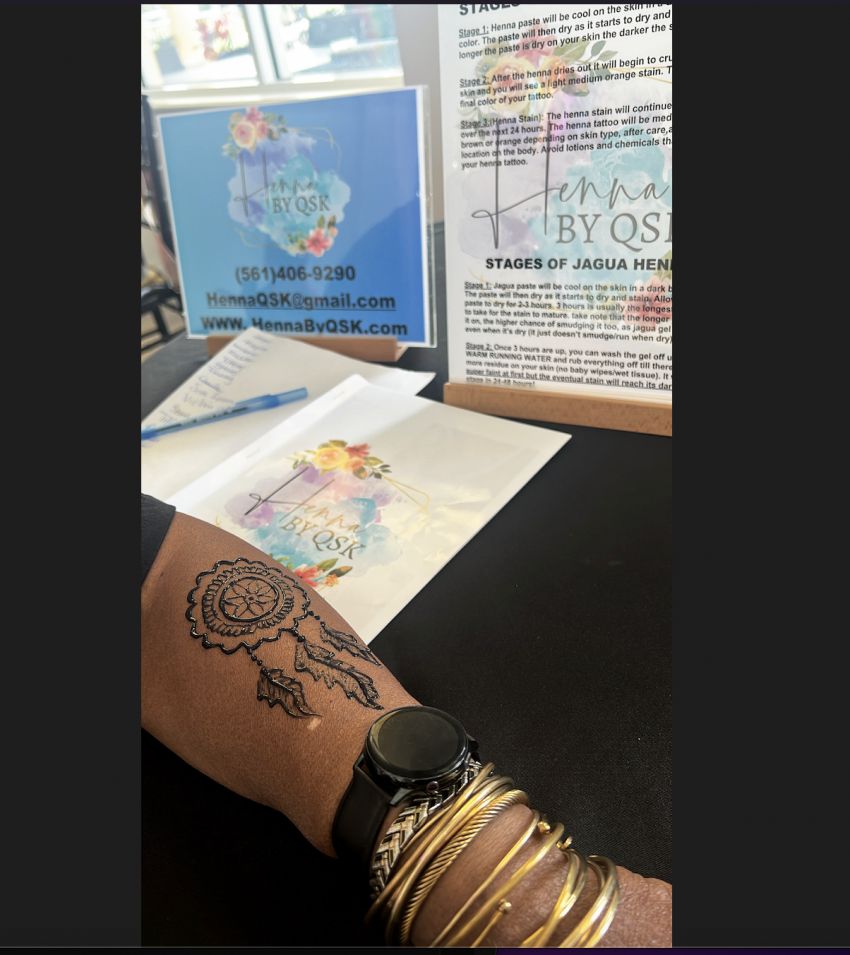The image displays the forearm of a dark-skinned individual adorned with a striking black tattoo resembling feathers or a feathered circle. The arm is accessorized with multiple gold bracelets and a black wristwatch, though the watch face is not visible. The background features an assortment of signs and papers, including a table with a blue pen and sheets of paper. Prominently displayed is signage reading "Henna by QSK," including a blue sign with contact information: "561-469-9290, hennaqsk@gmail.com, www.hennabuyqsk.com." Another white sign with black text provides further details about the henna offerings, though the text is too small to read. The upper left corner of the image reveals a window with sunlight streaming in, casting a bright yet indistinguishable view of the outside.